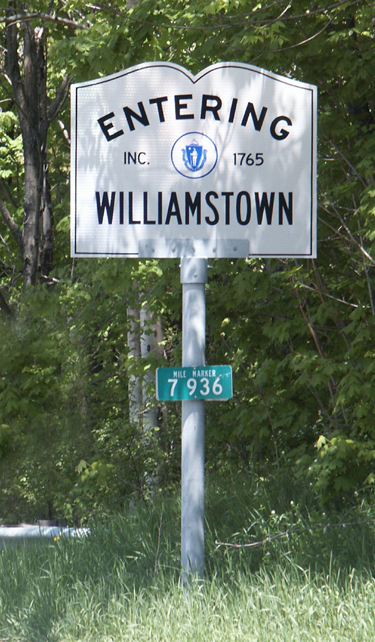This is a rectangular image depicting a welcoming sign for Williamston, established in 1765. The sign features a distinctive design with a heart-like curve at the top center while the rest maintains a square shape. Painted in silver with bold black text, the sign prominently reads "Entering Williamston" and includes a white and blue logo resembling a shield, though the detailed imagery on the shield is too small to discern clearly. Adjacent to the sign is a green mile marker with white text indicating "Mile Marker 7936." The background is a dense forest with a variety of trees, bushes, and unkempt grass, adding to the overall verdant ambiance of the scene. The untamed greenery, with its tall, wildly growing grass and overgrown trees, casts an inviting and natural atmosphere, making green the dominant color theme in the image.